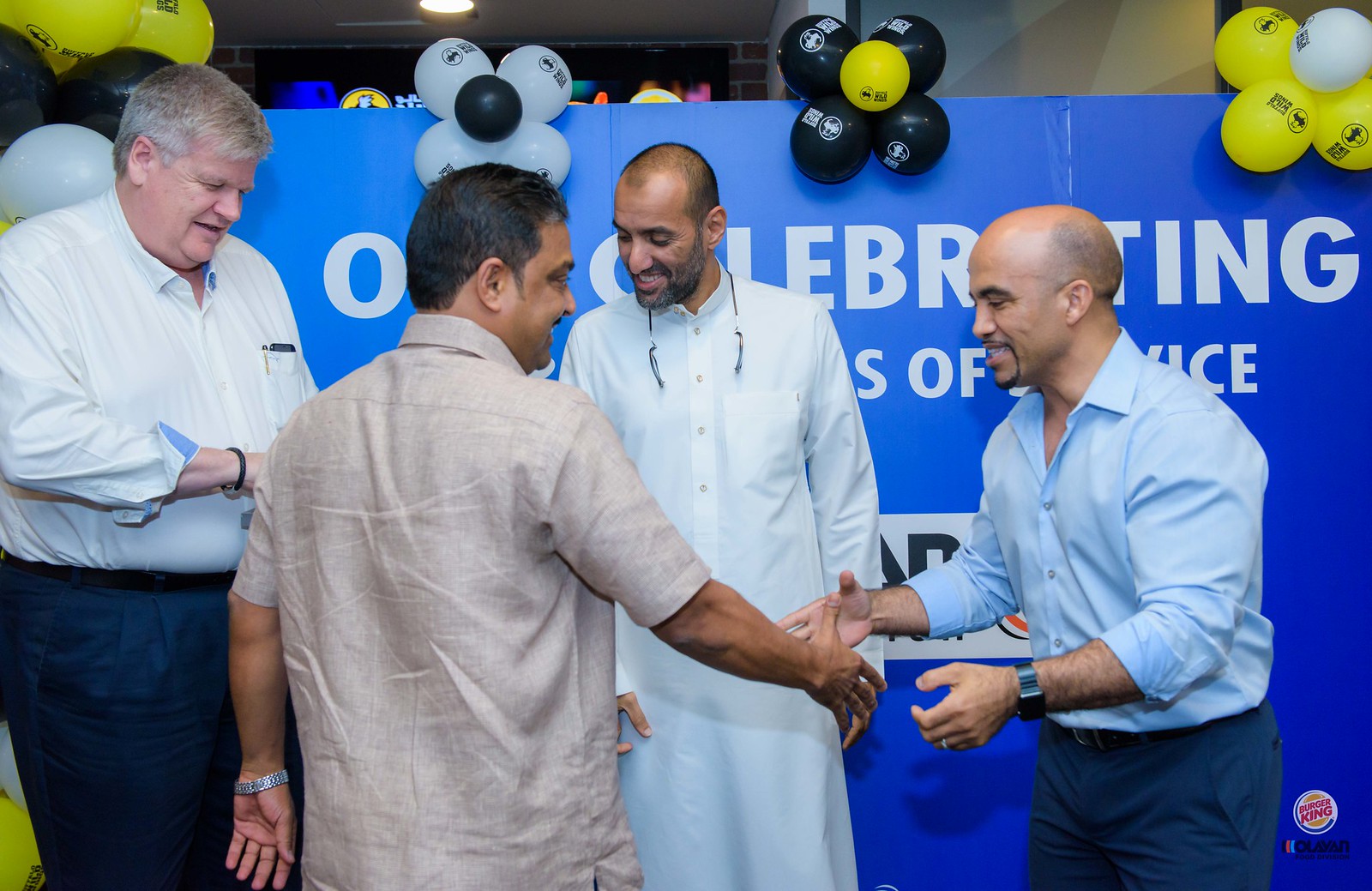In this color photograph, four men are standing in front of a large blue wall adorned with celebratory white text partially obscured by their presence. The word "celebrating" is discernible amidst the decorations, which also include black, yellow, and white balloons at the top of the wall. On the far left stands a tall, graying Caucasian man, dressed in a button-up long-sleeved collared shirt and dark blue pants, and he's facing rightward, looking downward. Next to him is a man in a tan, khaki-colored collared shirt with sleeves ending just above the elbows. He appears to be reaching over to shake hands with the third man, who is wearing a blue buttoned-up collared shirt with folded sleeves reaching a little over halfway up his forearms, and dark blue pants. This man is also the shortest in the group, bald, with a mustache and goatee, and he is sporting a watch. Behind them, a man in a white, ankle-length robe, resembling traditional Middle Eastern attire, gazes to the right. The diverse group seems to be part of a celebratory event, ostensibly linked to Burger King, given a faint logo in the background. The image reflects a moment of mutual congratulation and celebration.